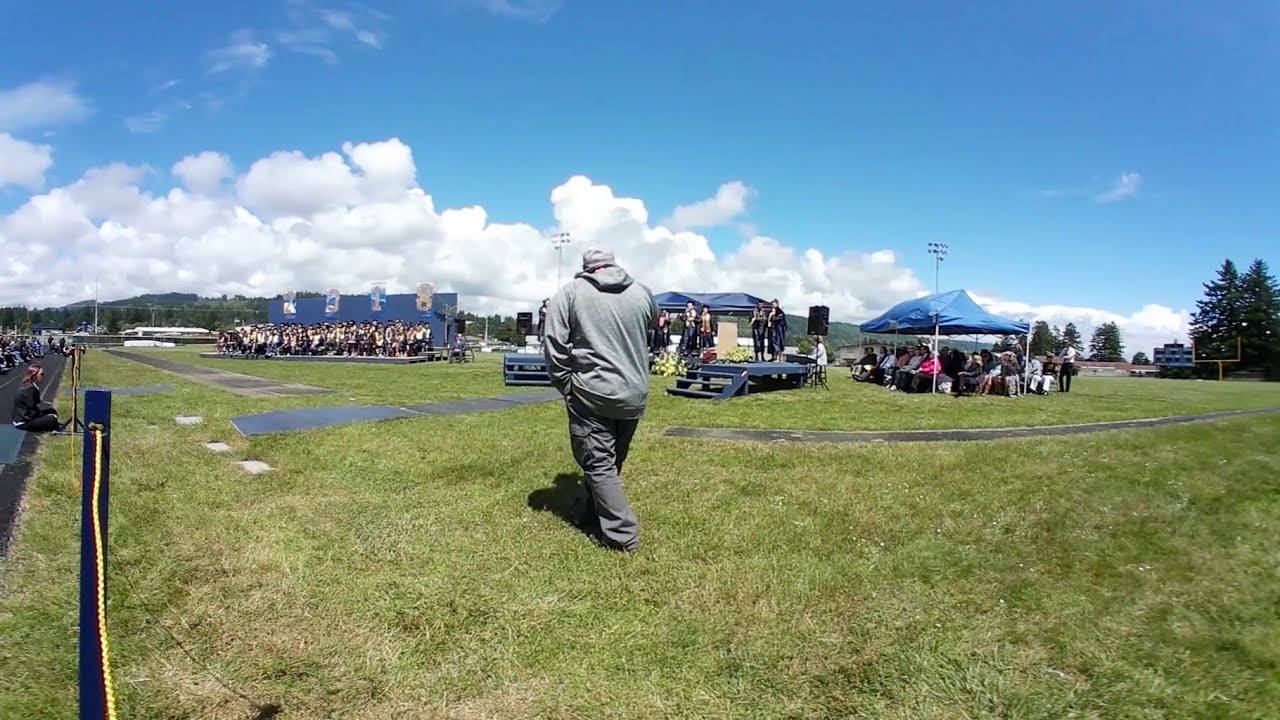The image depicts a burly, muscular man walking away from the camera on a grassy field under a partly cloudy sky. He is dressed casually in a gray cap, a thick gray hoodie, and olive-colored baggy jeans, which seem out of place for the event. The setting appears to be quite warm and sunny. The scene is lively, with many people gathered under blue tents facing a stage decorated with banners. The stage features several individuals who appear to be part of an orchestra or group performance, possibly a graduation ceremony. The central area of the photo is filled with people sitting and standing, creating a busy atmosphere. The overall setting suggests a public park or outdoor venue with a large crowd attending a significant event.